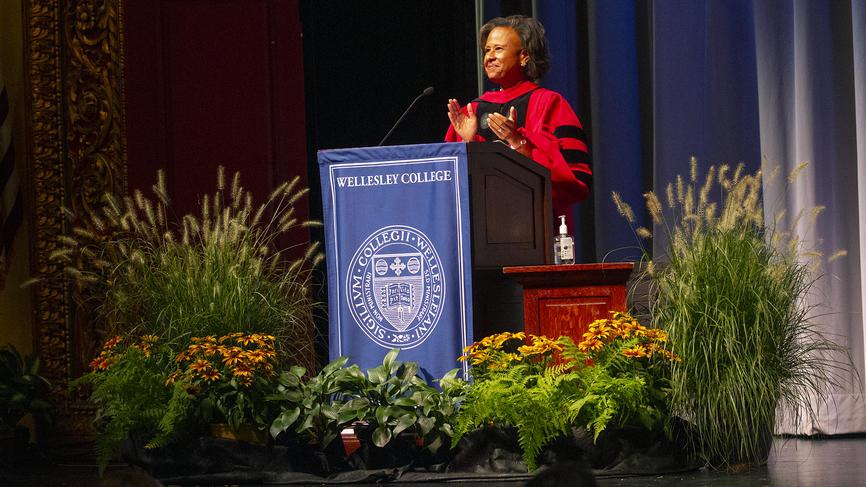The photograph captures a professor dressed in a distinguished red and black academic gown, standing at a dark brown wooden podium, either preparing to clap or already clapping her hands in apparent applause. She has a short brown haircut and is beaming with a bright smile as she engages with the audience. In front of the podium, which features a blue banner with the white-lettered insignia of Wellesley College, lies an array of potted plants, tall grasses, and flowering arrangements that add a touch of natural beauty to the scene. To the right of the podium, a small table holds a bottle of hand sanitizer. Behind her, floor-length white curtains stretch across the background, with one side of the image enveloped in darkness, suggesting a spotlight that focuses all attention on the speaker. The overall setting, accentuated by the blue banner and the ornamental plants, suggests a formal event, likely a graduation ceremony, taking place at Wellesley College.